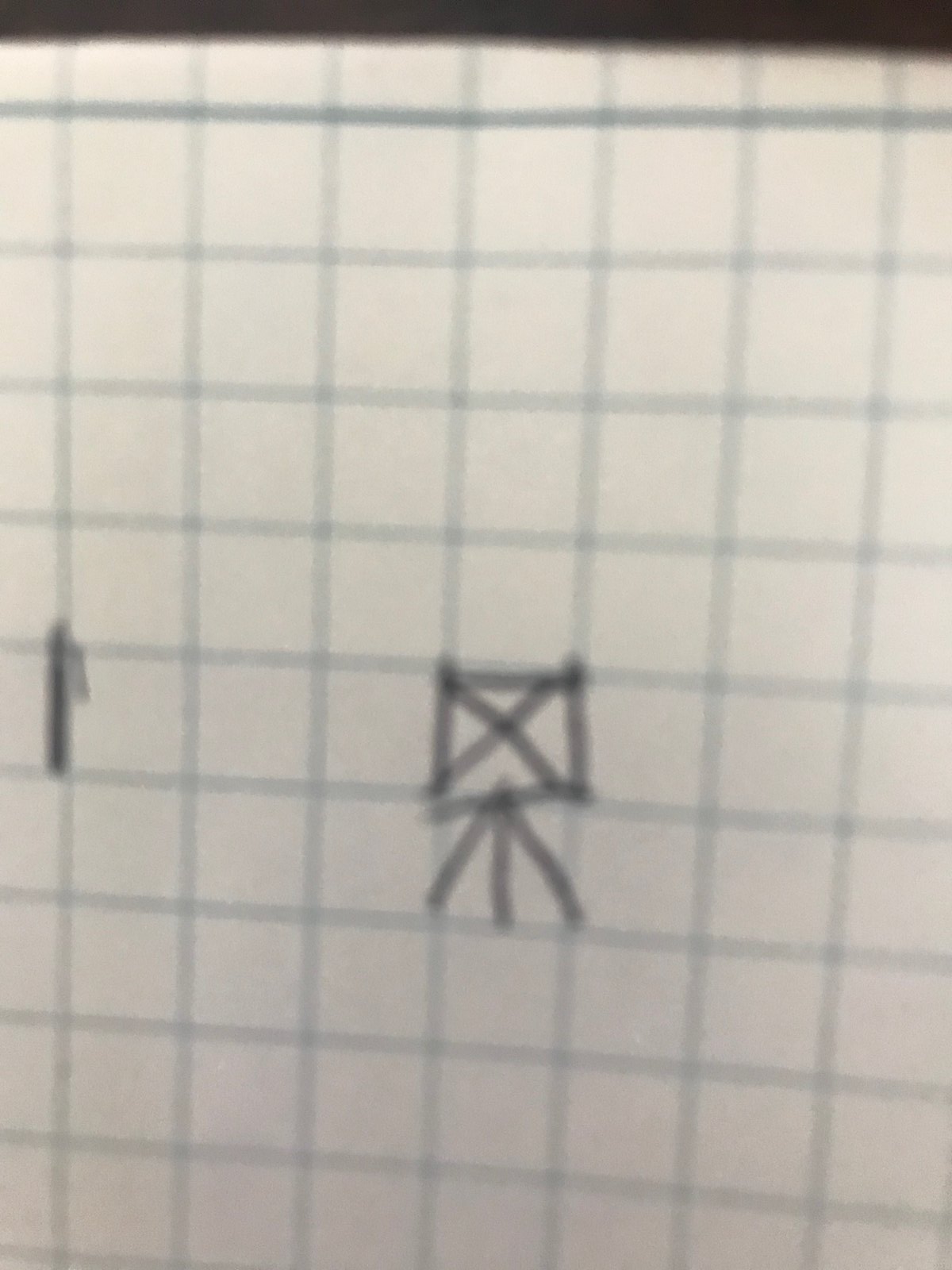This image depicts a book page with a pristine white background. The page is adorned with a grid of light blue lines, both horizontal and vertical, forming a tapestry of small squares. In the left margin, there is a tiny inscription in pen, resembling the letter "L." 

Within the grid, precisely three squares to the right of the initial "L," another square is meticulously drawn in black ink, superimposed over the blue grid lines. This black square features a central "X" intersected by additional lines that extend downward, creating a triangular arrangement resembling legs. There is also a central leg protruding from the bottom.

The rest of the page remains untouched with no additional markings or writings, maintaining a clean and uncluttered appearance. This description aims to capture the meticulous details and structured layout of the page with its subtle yet deliberate elements.